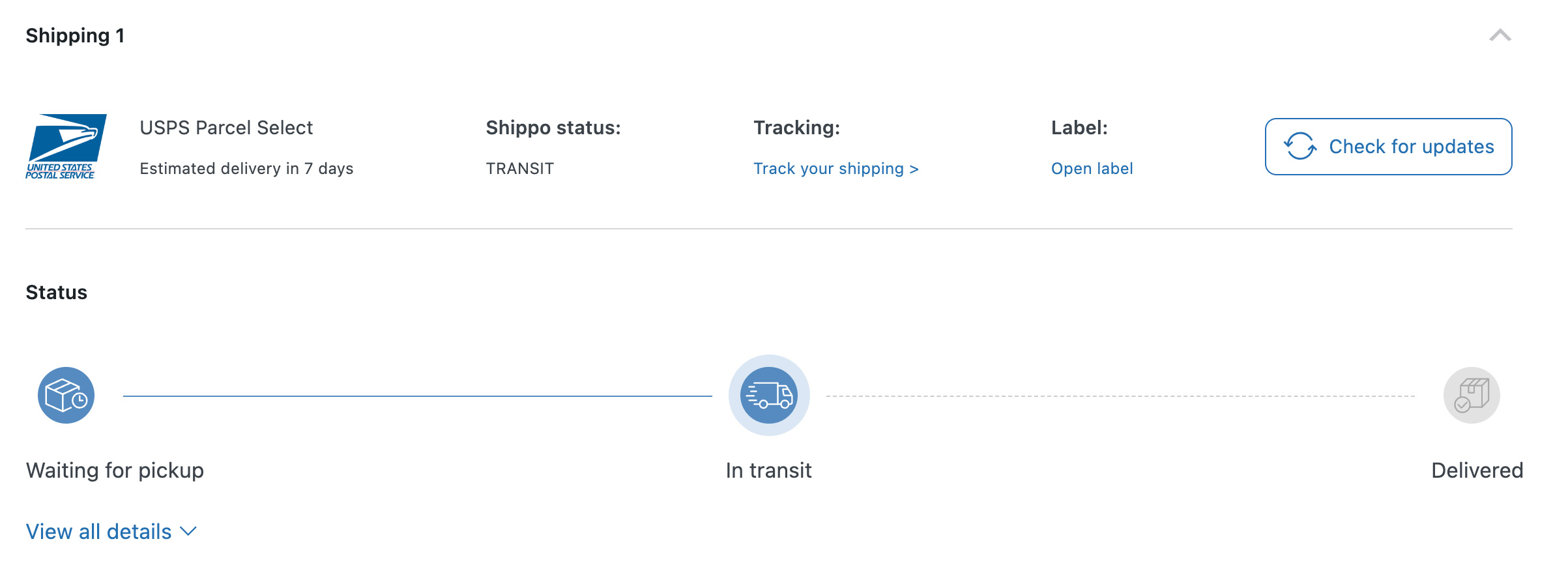In this screenshot, we are presented with a clean white background featuring various texts and icons related to a shipping service update. In the upper left corner, highlighted in dark blue text, is the heading "Shipping 1." Directly below this, the logo for the United States Postal Service (USPS) is prominently displayed in blue and white. Adjacent to the logo, it reads "USPS Parcel Select," followed by smaller text that states, "Estimated Delivery in seven days."

To the right of this information is a section labeled "Shippo Status" in bold text, with the current status, "Transit," written beneath it in smaller text. The next column over is titled "Tracking." Beneath this heading, in light blue text that likely functions as a hyperlink, is the phrase "Track Your Shipping."

Further to the right is another column labeled "Label," and under this heading is a button labeled "Open Label." Continuing further right, there is a white action button with the blue text reading, "Check for Updates."

Directly beneath the USPS logo, the section is labeled "Status" in dark black, bold text. Underneath this, there is an icon of a package enclosed within a blue circle, and immediately below this icon, it indicates the current status as "Waiting for Pickup."